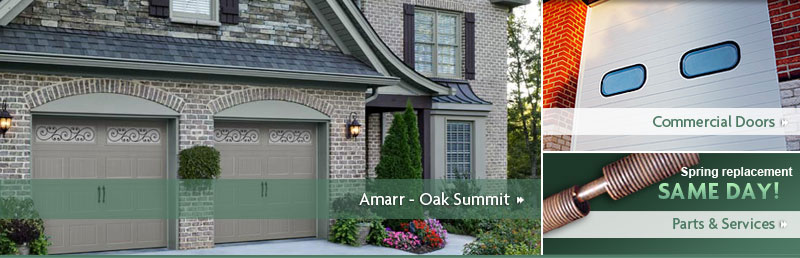The image consists of three distinct panels. The prominent left panel features a brick house with lighter-toned bricks and a black roof. The residence has two garage doors, adorned with surrounding shrubbery and flowers. A tall tree is visible at the side of the house, and the scene is set against a clear blue sky. Brown shutters frame the windows, and two lampposts are affixed to the garage. Notably, a green banner stretches across the garage doors, bearing white text on the right side that reads "Amarr-Oak Summit" in capital letters. 

On the right, two smaller panels are arranged vertically. The top panel showcases a section of red brick siding and a white garage door with two black-trimmed oval windows. This panel includes a white banner featuring green text that states "Commercial Doors," with the 'C' and 'D' capitalized.

The bottom panel presents a green background illustrating a set of springs. Overlaid on this background is text advertising "Spring Replacement," followed by "same day parts and services," emphasizing prompt and reliable service.